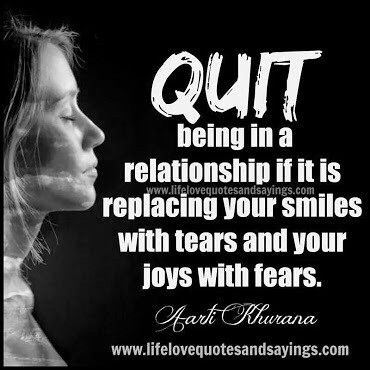The image features a striking black-and-white photograph combined with graphic design and bold typography, typical of an inspirational message seen on social media. In a square format, the left side prominently displays a young woman in profile with short, wispy hair, her eyes closed as if she is contemplating or feeling sad. The background is black, enhancing the contrast and making the white and gray tones of her face more striking. An added special filter gives her face an ethereal, cloudy effect.

The center of the image displays the primary text in a strong, bold style: "QUIT being in a relationship." Underneath, in lowercase letters, the text continues, "if it is replacing your smiles with tears and your joys with fears." At the bottom of the quote, in a lighter script, the author is credited as Ardy Karana. Also in light script at the bottom edge of the image is the URL "www.lifelovequotesandsayings.com."

The overall design blends the solemn, reflective portrait of the woman with the powerful, motivational message, emphasizing the theme of prioritizing one's emotional well-being over a detrimental relationship.